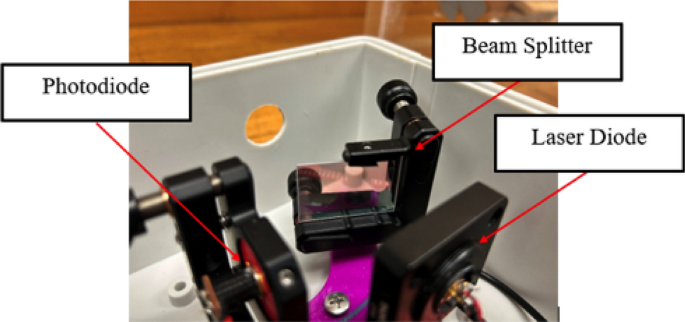This image showcases a detailed view of laboratory equipment enclosed in a white or light gray box, situated against a wooden background. The interior houses three distinct black electronic devices, each securely mounted and connected with visible wiring. The equipment includes a photodiode, which is labeled within an oblong white box with black printing, located on the left. To the right is a beam splitter, identifiable by its black body featuring an area that appears pink or copper. Below the beam splitter, at the bottom right, is a laser diode, also labeled clearly. Red arrows point down toward these devices, guiding the observer through the setup and indicating various parts of this experimental or technological interface. The equipment and its layout suggest a sophisticated assembly within a laboratory setting, likely for precise optical or laser-based experiments.